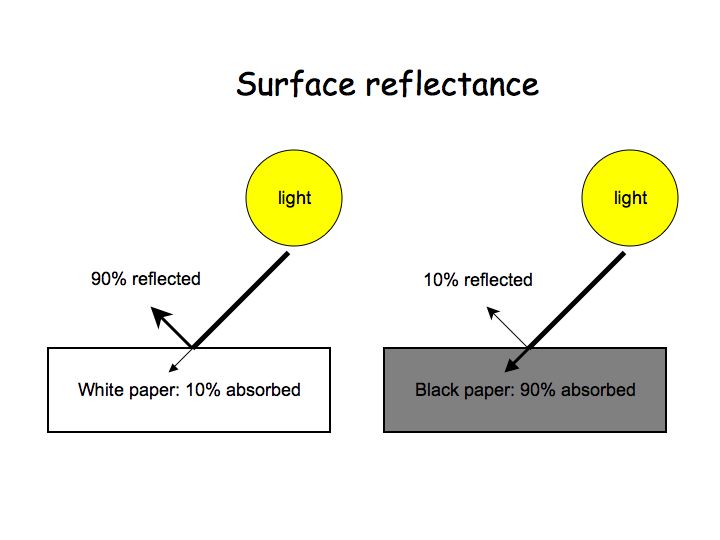The diagram on a white background is titled "Surface Reflectance" in bold black text at the top. It is divided into two halves, each illustrating the behavior of light when it interacts with different surfaces. On the left side, there is a depiction involving a yellow circle labeled "Light". An arrow from this circle hits a white rectangular area, bordered by a thin black line and labeled "White Paper." The annotations indicate that 90% of the light is reflected, while 10% is absorbed. On the right side, a similar yellow circle labeled "Light" directs an arrow towards a gray-shaded rectangle labeled "Black Paper." Here, the diagram notes that only 10% of the light is reflected, and 90% is absorbed. This visual comparison effectively illustrates the difference in light absorption and reflection between white and black paper.